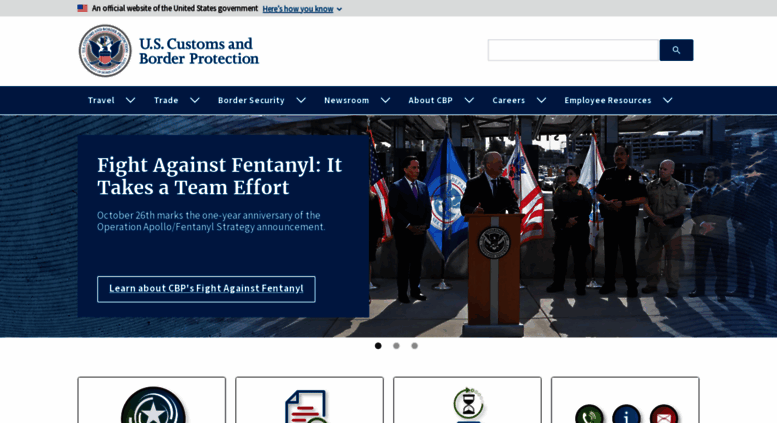In this image intended for a government web page, the top banner is grey with the American flag prominently displayed in the top left corner. Next to the flag, in black font, it states "An official website of the United States government," accompanied by blue text reading "Here's how you know" with a downward-facing arrow. Adjacent to this, the U.S. Customs and Border Protection (CBP) seal is displayed, featuring the organization's name in blue font beside it.

To the right of the banner is a search box with a white search icon set against a blue background. Below the main banner, a secondary blue banner with white text features various dropdown menu options: "Travel," "Trade," "Border Security," "Newsroom," "About CBP," "Careers," and "Employee Resources," each followed by a downward-facing arrow.

Beneath this, a green background with a blue box displays white text that reads: "DHS Fact Sheet: President Proclamation to Suspend and Limit Entry and Joint DHS-DOJ Interim Final Rule to Restrict Asylum During High Encounters at the Southern Border." Following this header, a white square with blue text prompts users to "Read the Fact Sheet."

The US Customs and Border Protection seal appears again, characterized by a grey outline, a white background, blue lettering, and a blue eagle with stars and red stripes. Below the eagle, the text reads "Department of Homeland Security."

At the bottom of the image are five circles, each containing different icons:
- The first and darkest circle contains a white star within a grey circle.
- The second circle contains a page with red lines and a green circle with a black check mark.
- The third circle features a grey hourglass.
- The fourth circle contains three black circles, with the first inner circle being green with a white phone icon, the second being blue with a white eye icon, and the third being red with a white envelope icon.

This detailed description encapsulates the various visual elements and textual content of the government web page image.